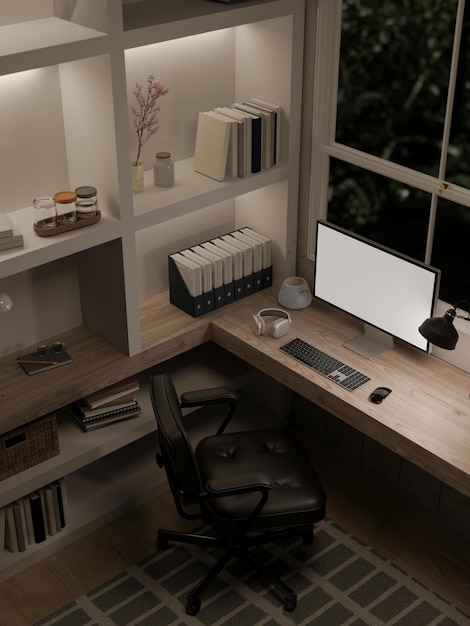This overhead image captures the intimate detail of a home office corner, taken from a ceiling perspective. The centerpiece is a light brown, cushioned desk chair with black legs and armrests, empty and poised in front of an L-shaped wooden desk. The floor underneath features a distinctive brown carpet with dark brown square patterns that form a grid over light wood hardwood flooring.

On the desk, a white-screen computer monitor catches the eye, positioned against a nocturnal backdrop visible through a white-framed window, with faint outlines of leafy foliage outside. Accompanying the monitor are a black keyboard and mouse, as well as a pair of white headphones.

To the left of the chair, a spacious white bookcase stands with three prominent cubbies. The lower cubby houses an assortment of books, while the middle shelf displays three glass jars with colorful lids. The upper cubby features a row of books laid flat beside a small plant. Directly adjacent to this bookcase, beneath the desk, is an additional storage area with more books and notebooks arranged haphazardly.

A black lamp emerges slightly from the desk scene, casting light across the workspace. The visual coherence of the office setup is underscored by the thoughtful organization of books and personal items, set against the neatness of the wood and white-themed furniture. The whole composition gives a warm, functional yet cozy ambiance, accentuating the quiet productivity of a personal workspace at night.